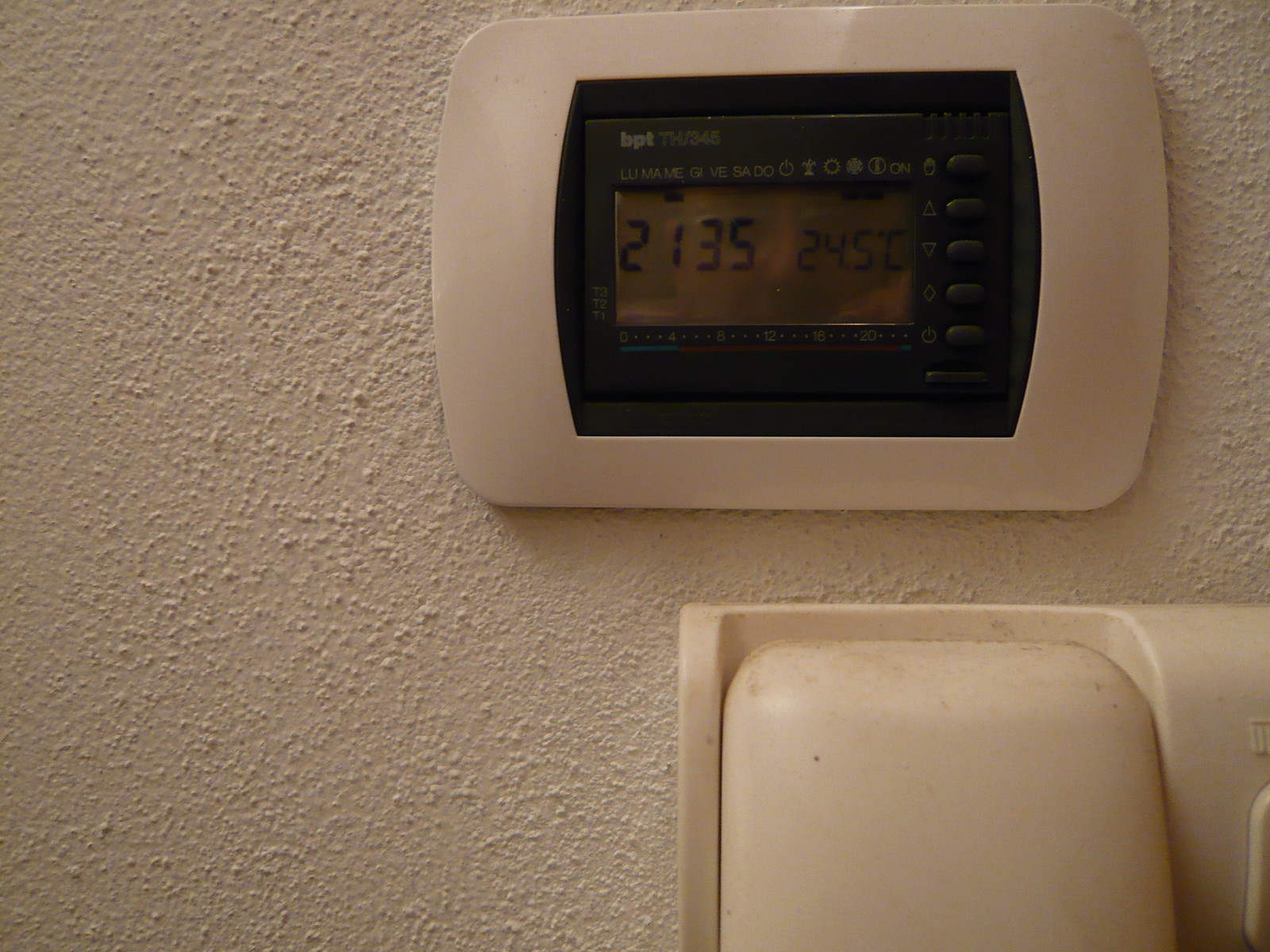This photograph, taken inside a building or house, focuses on a wall-mounted thermostat and a section of a plastic handheld phone. The wall features a light rose-colored, textured surface that sets a subtle background for the objects.

In the bottom right of the image, the upper part of a wall-mounted, off-white plastic phone handset is visible. The handset rests in its cradle, showing signs of wear and dirt marks, suggesting it has been in use for a considerable time.

Above the phone, a sleek white oval shape frames a black, almost square, digital thermostat. The thermostat displays the current time "21:35" and the temperature "24.5°C" prominently. Below the display, a blue and red line indicates temperature settings, accompanied by six buttons aligned vertically on the right: a large, rectangular gray button at the bottom and five oval-shaped buttons above. These include controls likely for power, heating, cooling, and temperature adjustments, though some labels are partially obscured. At the top of the thermostat, the make "BPT" and model number "TH/345" are clearly printed, identifying the device.